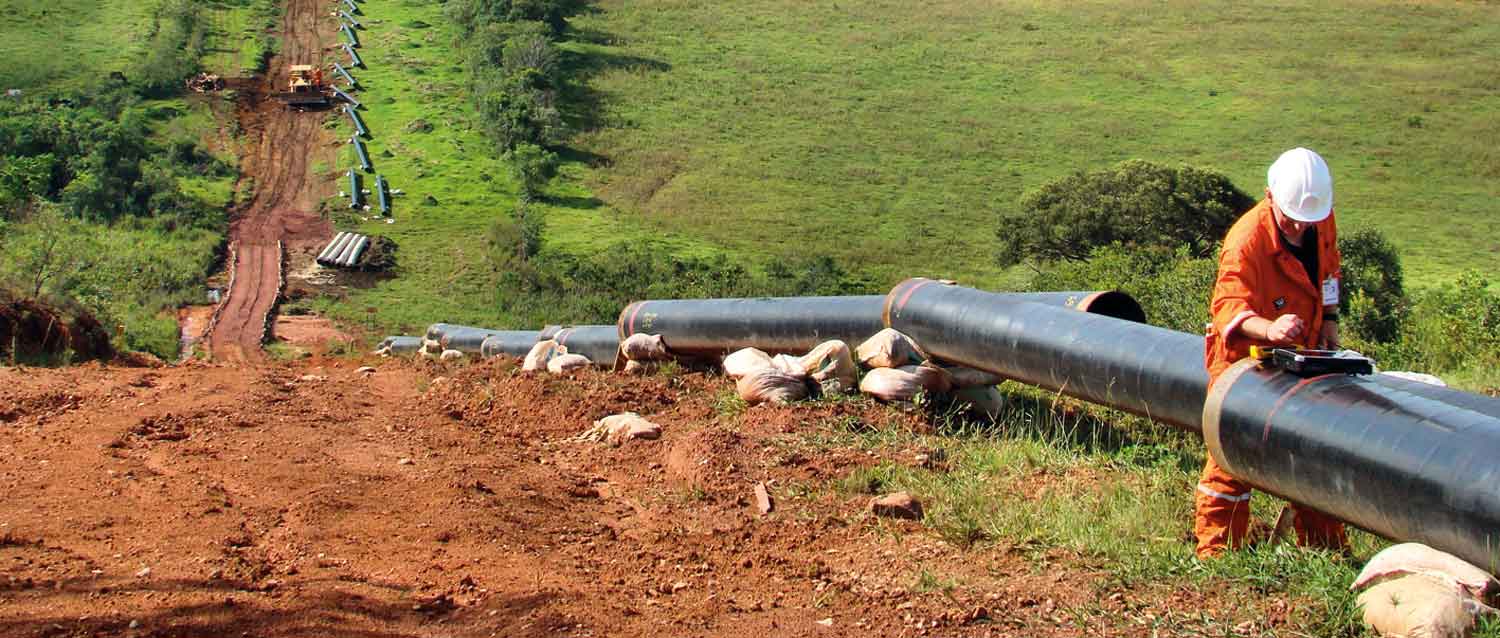A detailed scene of a construction site shows a worker in an orange jumpsuit and white construction hat standing at the right edge of the image, overseeing the assembly of large black pipes. The worker, positioned at the beginning of a pipeline section, appears to be handling a piece of equipment or box on the pipe, perhaps used for connecting the sections. The pipeline, which is composed of unconnected segments resting on light-colored sandbags, descends down a carved path on a green hillside. Surrounding the construction work are lush green fields and trees. In the upper left corner, a yellow piece of machinery, possibly a backhoe or plow, is visible near a red dirt road that stretches from the corner to the lower third of the image.